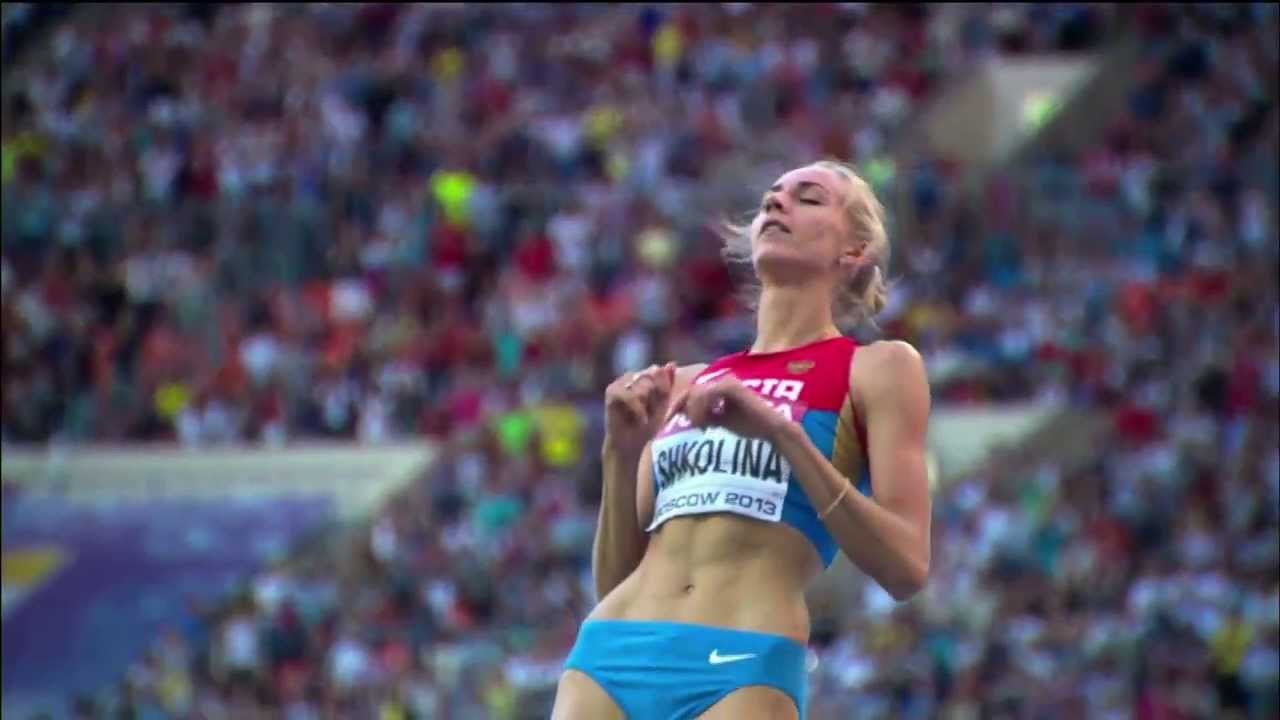The image depicts a female track and field athlete, captured in an Olympic event in Moscow, 2013. The athlete, whose name tag reads "Kolina," wears a sports bra that is blue and red, and light blue Nike spandex shorts. She has a fair complexion and blonde hair. Positioned slightly off-center in the photograph, she appears to be stretching or leaning back with her eyes closed, possibly catching her breath after an intense run. In the background, a massive crowd fills the stadium, although they are blurred to maintain focus on the athlete who is in remarkable physical condition.